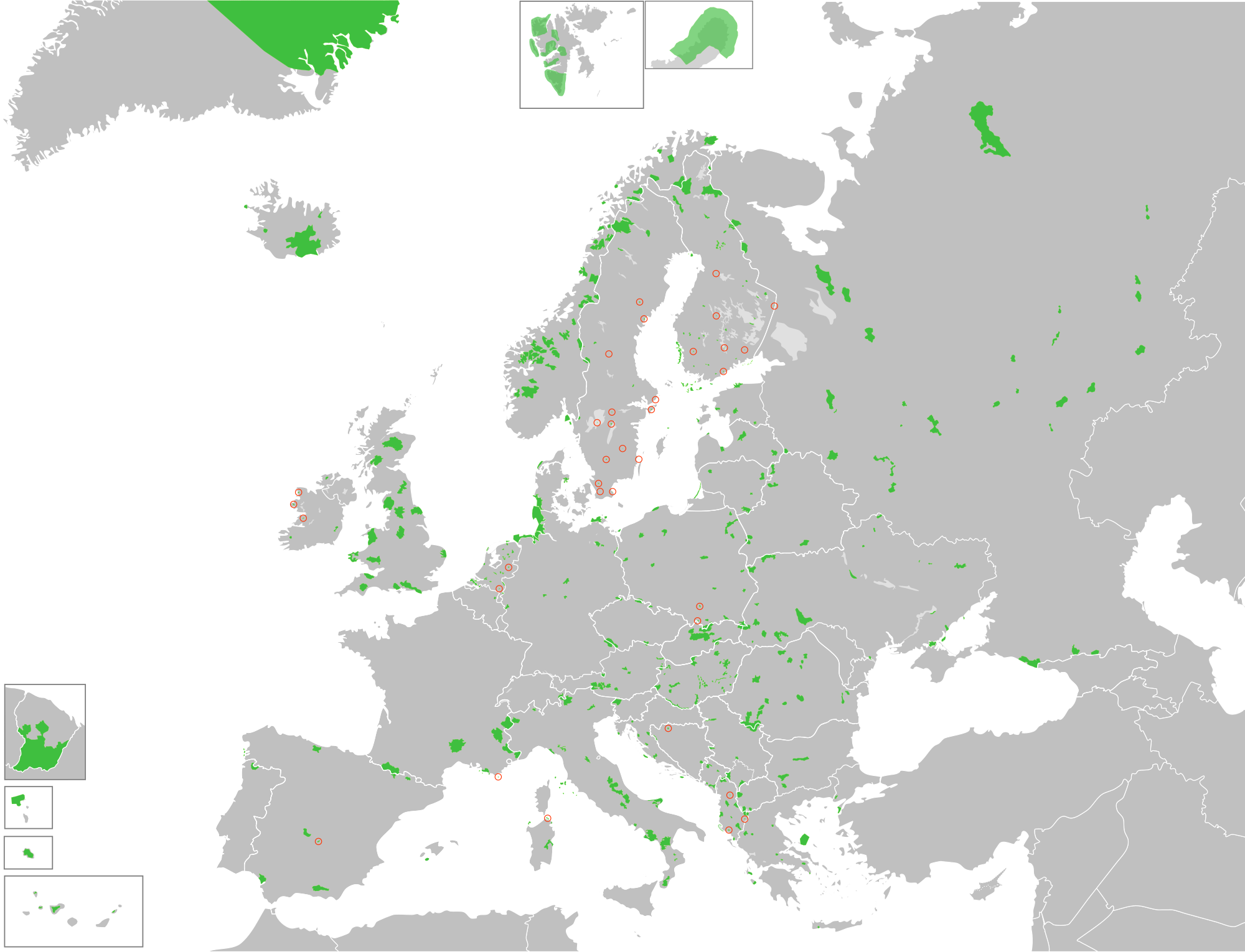This image depicts a detailed map focusing on the continents of Europe and Asia. The map uses a stark color contrast, with the water bodies rendered in white and the landmasses in shades of grey. Each country's borders are clearly delineated with white outlines, highlighting their shapes. Scattered across the map are various spots marked in a vibrant grass green, though their significance is unclear. Additionally, numerous hollow red circles are dispersed throughout the map, yet these also lack any explanatory context.

At the top center of the map, a distinct square section features more land delineated with patches of green. Directly to the right of this square is a rectangular area, similarly exhibiting grey land overlaid with green patches. In the lower left corner, there's a vertical rectangle predominantly in grey, outlined in white, with the upper half filled in green. Below this are two smaller boxes, completely filled with green. At the very bottom of the image, a horizontal rectangular box displays several islands, some grey and some green, adding further detail to the map's intricate presentation.